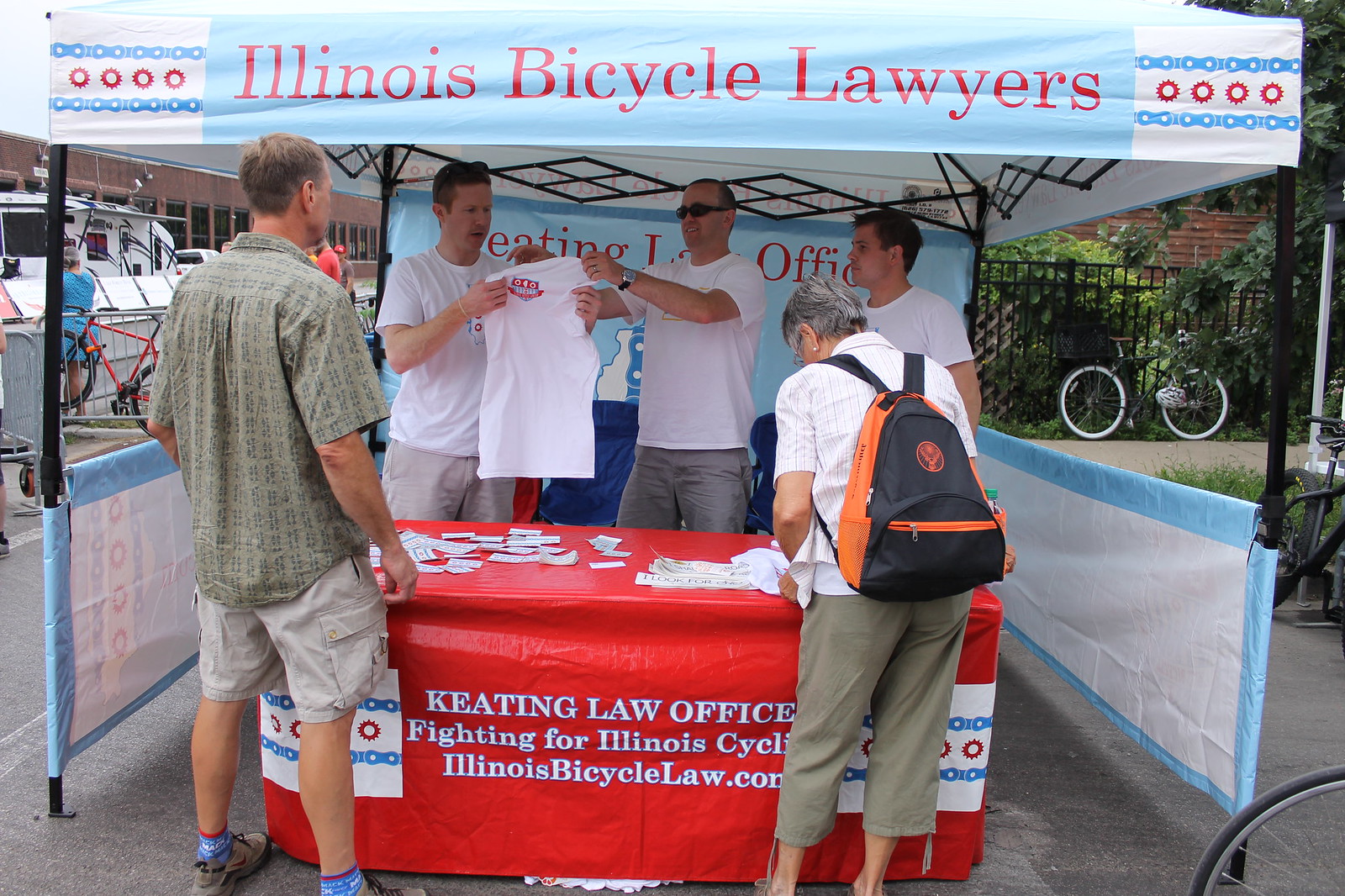The image depicts an outdoor promotional booth for "Illinois Bicycle Lawyers" at an event that resembles a job fair. The booth, which is covered by a collapsible light blue tent with red lettering, features branding elements such as a bicycle chain graphic and red sun symbols. Three white men, all dressed in white shirts and light gray or beige pants, are stationed behind a table with a red tabletop bearing the text, "Keating Law Office, Fighting for Illinois Cyclists, IllinoisBicycleLaw.com" in white lettering. They are holding up white t-shirts, possibly displaying the Illinois Bicycle Lawyers emblem. In the foreground, a white man and woman, with the woman carrying a black and orange backpack, are seen from behind, engaging with the booth and examining business cards or other informational materials. Additional context includes a bicycle parked against a fence, a small boat or yacht partially visible to the left, and a building in the background.